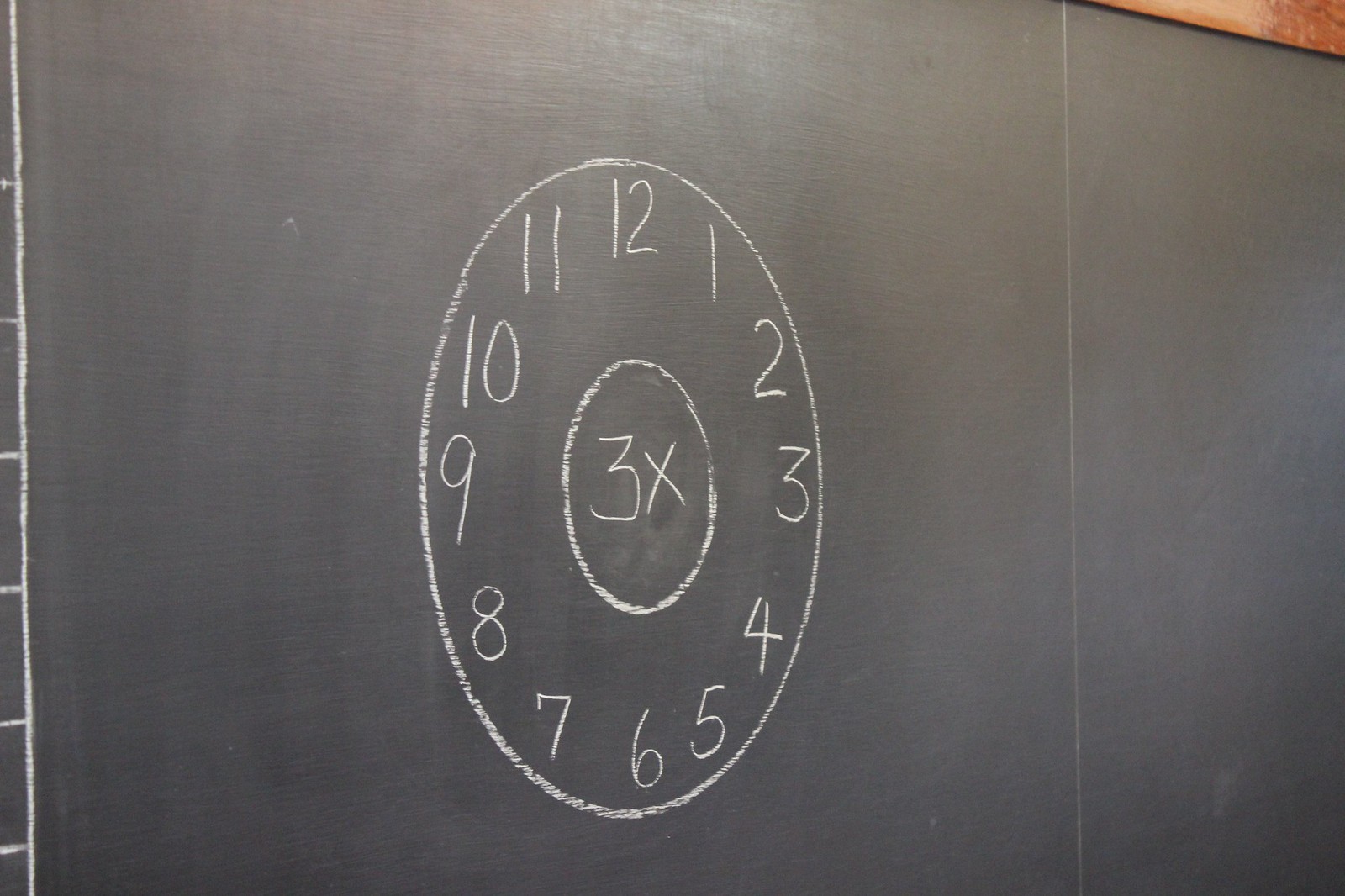This image features a large, black chalkboard set into a wooden frame, with a neatly drawn clock face using white chalk. The clock face consists of two concentric circles: a larger outer circle containing neatly written Arabic numerals from 12 to 11, clockwise, and a smaller inner circle that features the inscription "3X." Despite some ambiguity around the meaning of "3X," the overall appearance suggests a clock. Additionally, there are white chalk lines along the far left edge of the chalkboard and a vertical line on the right. The chalkboard's surface appears mostly clean, with subtle gray markings and a small brown bar across the top right corner. White lights illuminate the setting, enhancing the clarity of the chalk drawing.